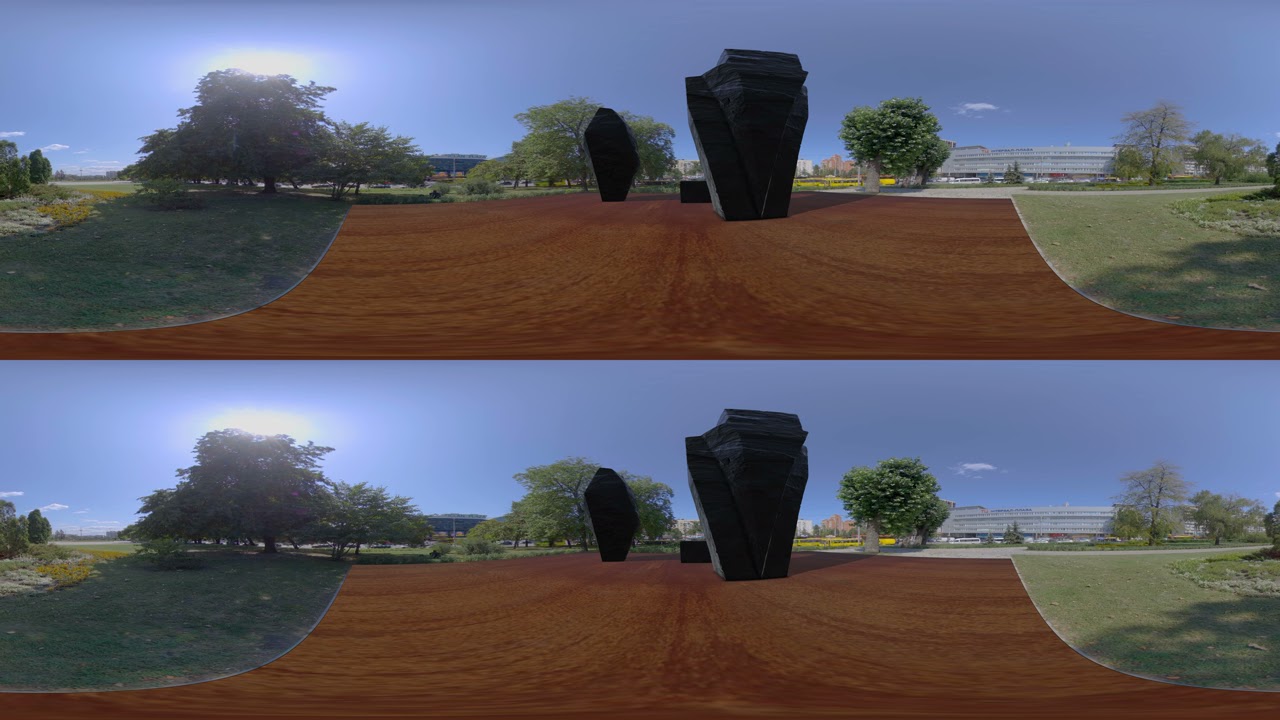The image depicts a park-like setting captured from a wide-angle perspective, featuring two horizontally stacked pictures taken seconds apart. At the center lies a well-manicured dirt patch, surrounded by patches of grass on both flanks. Prominent within this dirt area are three large rock formations of varying shapes: one resembles a block, another has a V shape, and the third tapers to an angled point on the right side. The rocks, predominantly black in color, appear to create a monument or sculpture-like arrangement.

Surrounding this installation is a lush environment characterized by tall, bushy trees that reach approximately 30 feet high, and manicured grassy areas. In the top right corner of the photograph, a building can be observed, adding to the park-like and somewhat urban ambiance. The sky overhead is mostly clear with a singular cloud, suggesting it is a bright, sunny day. The colors in the image range from the earthy tones of brown and tan of the dirt, to the verdant greens of the grass and trees, contrasted against the blue sky and the black and gray of the rock formations. There is no text visible in the image, emphasizing the natural and serene setting portrayed.